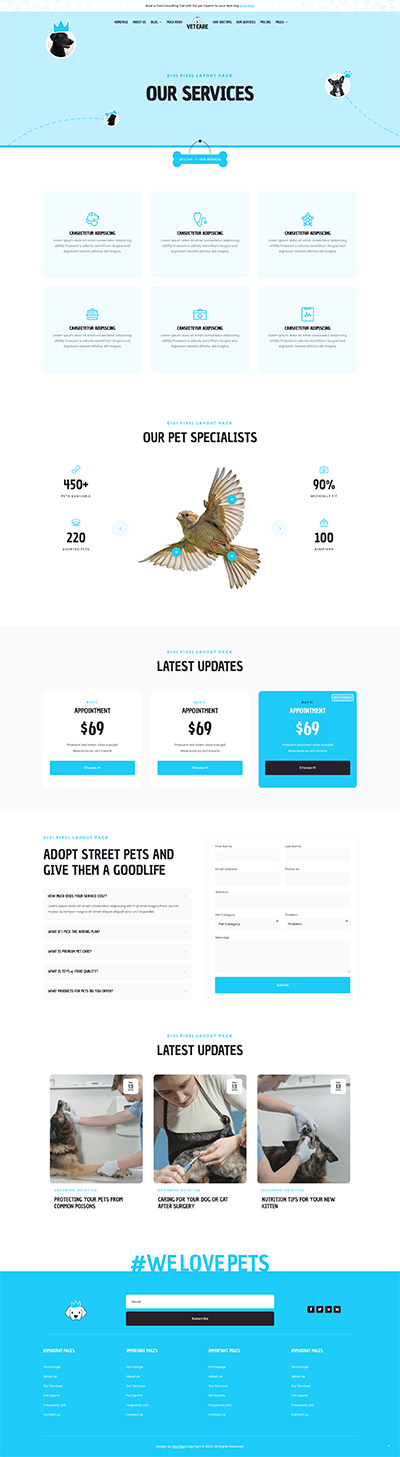Here is a cleaned-up and detailed caption for the described image:

---

This image features a veterinarians' website by VetCare with various design elements and sections. The top of the page is adorned with a light baby blue banner that reads "Our Services" in black lettering. The website has two prominent dog graphics: one to the upper left wearing a crown and another to the right.

Beneath the banner are six menu options, each contained in individual boxes, though the text is unintelligible due to low resolution. In the middle section, there is a section titled “Our Pet Specialist,” featuring an illustration of a bird with three blue dots on its wings and tail. Beside the bird, several statistics are displayed, including numbers such as 450, 220, 90%, and 100.

Further down, the "Latest Updates" section provides information on appointment prices, uniformly listed as $69, except for one entry highlighted in blue with a black button, contrasting the standard white background and blue buttons of the other entries.

The website also promotes pet adoption with a call to "Adopt street pets and give them a good life," alongside a locator tool for adoption services. Below this, additional updates focus on topics like protecting pets from poisons, postoperative care for dogs and cats, and nutrition tips for new kittens, although oddly, the image associated with nutrition tips shows a dog.

At the very bottom, the phrase "WeLovePets" appears in blue lettering. There’s also a search bar surrounded by various other menu options, all situated within a blue box but largely unreadable due to low resolution.